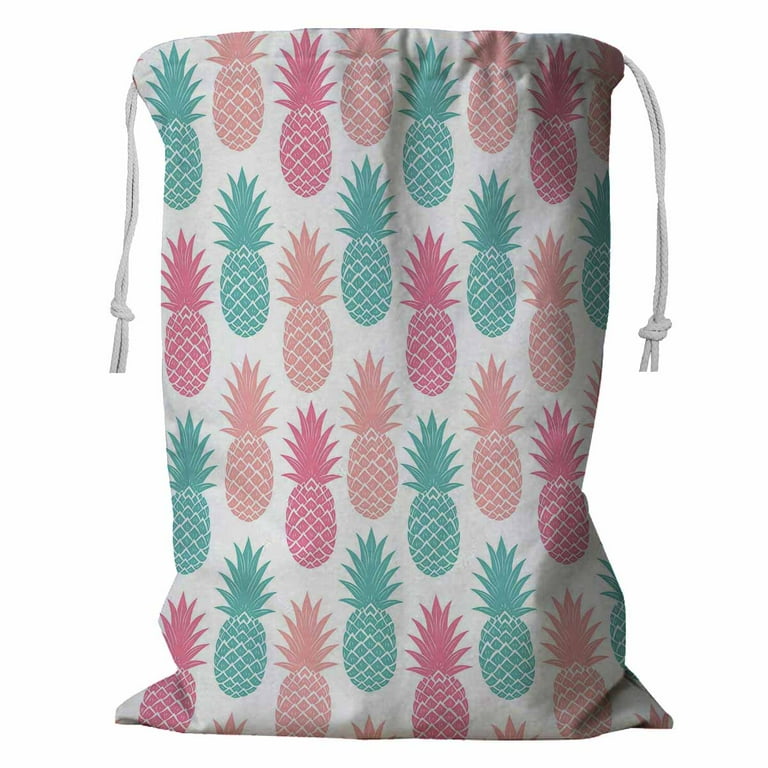This product image, likely intended for an online retail site such as Amazon or eBay, showcases a medium-small cloth drawstring bag against a completely white background. The bag is crafted from a whitish-gray cotton material and features a functional drawstring closure with two strings on each side, ending in knots. The bag's exterior is decorated with an array of small to medium-sized pineapples, printed in a variety of vibrant colors including bluish-green turquoise, peach, and pinkish-red. The pattern comprises approximately 30 pineapples, artfully arranged in a mixed-up fashion, creating a lively and playful aesthetic. The bag appears to be filled with an item substantial enough to allow it to stand upright in the photograph.